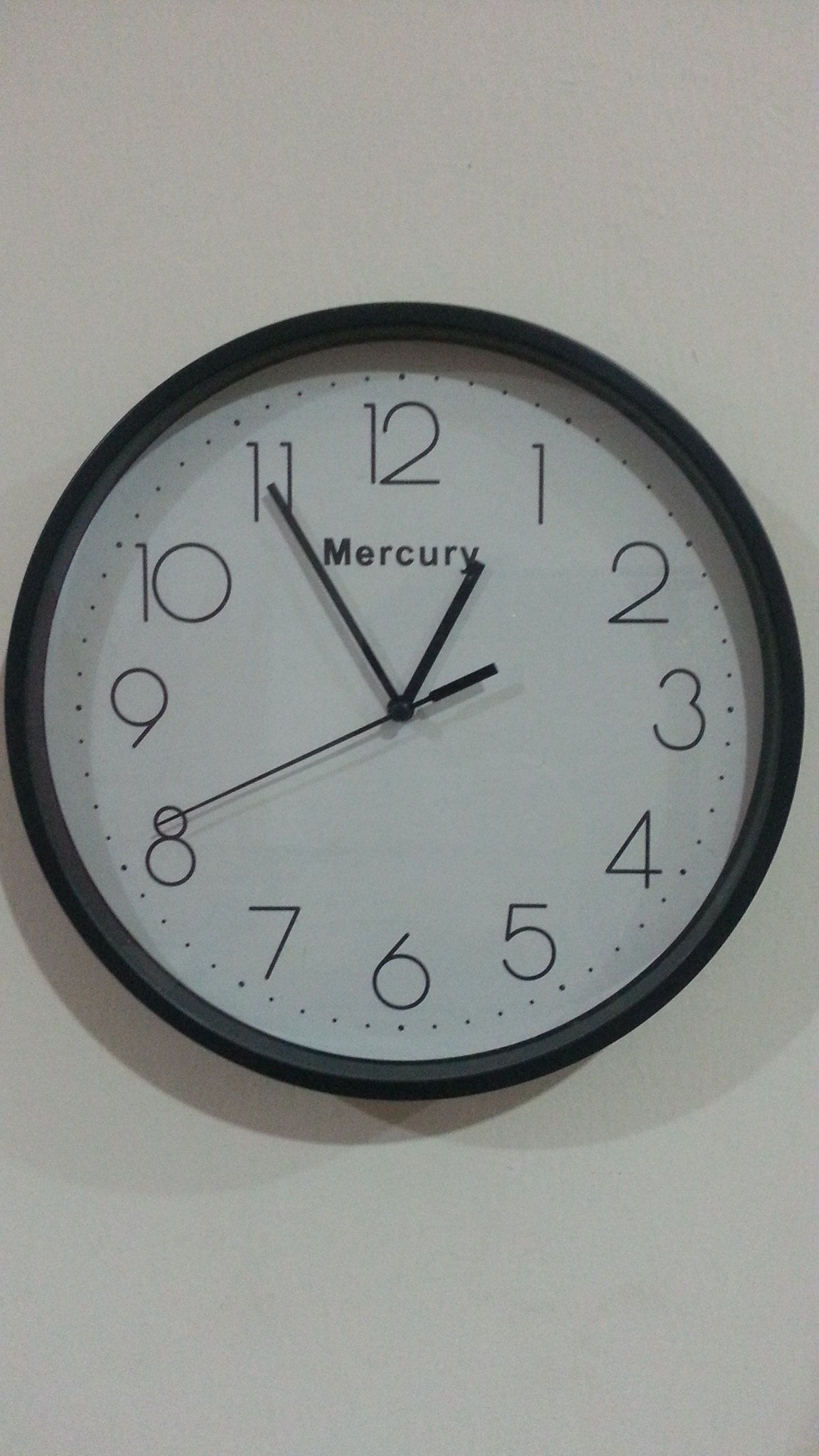The image features a round wall clock mounted on a white or off-white wall. The clock is encased in a black housing, which appears to be made of plastic. The front of the clock is covered by a flat, translucent panel that seamlessly connects to the housing. The clock face is white with bold black numerals and hands indicating the seconds, minutes, and hours. Beneath the 12 o'clock mark, the word "Mercury" is printed in black. Minute increments are denoted by small dots between the numbers. The clock displays the time as 12:55, with the second hand pointing at the 8, on the verge of advancing to the next minute.